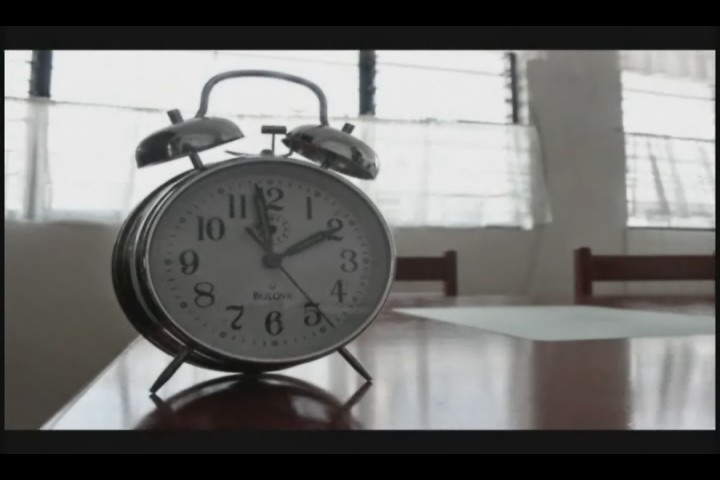This rectangular, black and white photo captures an indoor scene, focusing on an old-fashioned silver alarm clock with two round metallic bells on top, reminiscent of cymbals. The clock sits prominently on a shiny brown wooden table. The clock face, encased in glass or plastic, displays the numbers 1 through 12 in a clockwise manner. The minute hand is pointing at the 12, the hour hand at the 2, and the second hand is at the 5. The brand name "BELOVA" is visible above the number 6 on the clock face. Behind the clock, a piece of paper lies on the table, and further back, two chairs are tucked neatly under the table. The background reveals a white wall adorned with a row of windows featuring horizontally slatted coverings. The bottom half of each window has thin, translucent curtains, allowing daylight to stream in, suggesting that it is two o'clock in the afternoon.